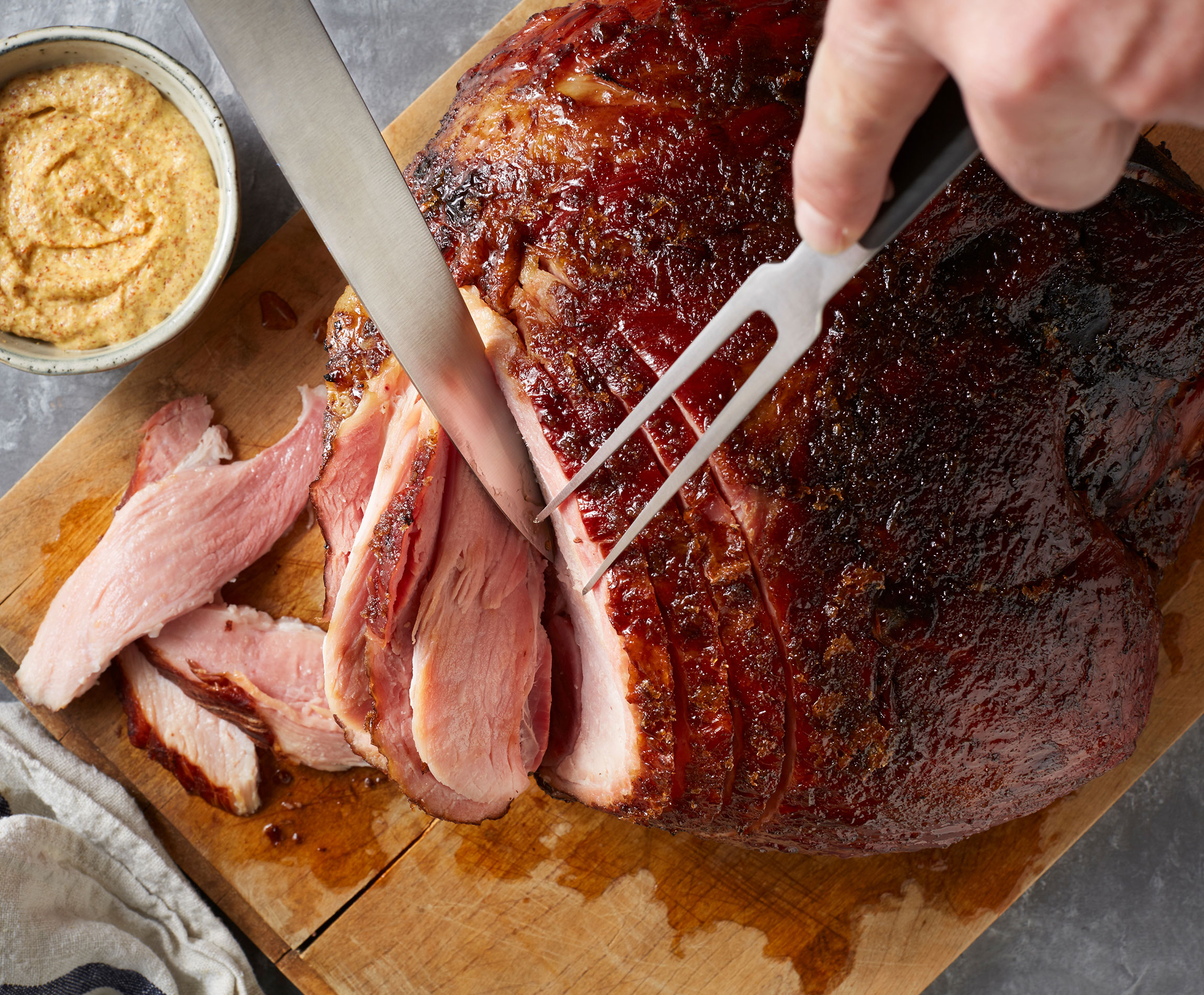This full-color photograph captures a tantalizing scene of a Caucasian man slicing a quarter ham on a well-used wooden cutting board, which shows dark stains from the meat's juices and a few splits along the edges. The ham appears to be expertly cooked and looks very delectable, almost glistening under the light. He wields a long knife in one hand and a fork in the other, carefully cutting into the meat. The angle of the photograph suggests it was taken from above, giving a clear view of the action. To the side of the cutting board, there is a small white bowl containing a yellow dipping sauce, likely mustard, adding a pop of color to the otherwise muted background. Additionally, a dish towel is casually laid next to the cutting board, emphasizing the casual yet engaging culinary moment.